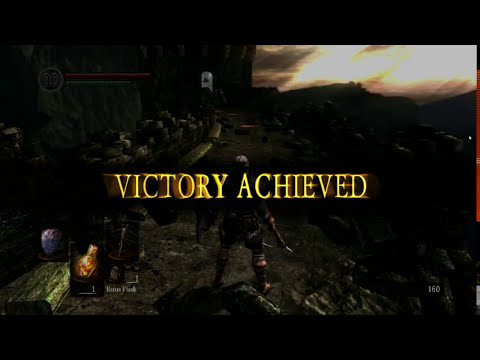In this dimly-lit screenshot from a third-person video game, the words "VICTORY ACHIEVED" are prominently displayed in glowing yellow capital letters in the center, signaling the aftermath of an epic battle victory. The focal point of the image is a Spartan-like character resembling Kratos from "God of War," equipped with a sword in his right hand and a shield in his left, dressed in a traditional Spartan outfit with boots. He is standing amidst a rugged, rocky terrain that extends to the far left, while the background features a mountainous landscape under a sky visible in the far right horizon, partially illuminated as if by distant sunlight. The bottom left corner displays various in-game icons and a mini-map, indicating vital gameplay elements, while a faint health bar and energy bar appear at the top of the screen.